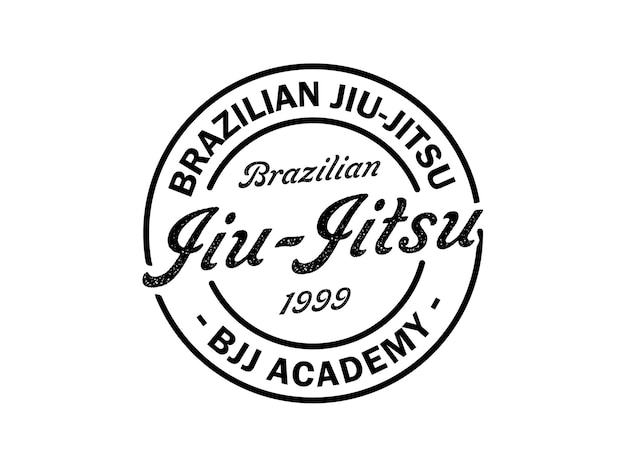The image depicts a black and white circular logo, reminiscent of an ink stamp. Against a plain white background, the outer edge of the circle features the phrase "Brazilian Jiu-Jitsu" at the top and "BJJ Academy" at the bottom in bold, capital letters. Inside the border, another smaller circle highlights the text "Brazilian Jiu-Jitsu 1999" in a sophisticated, calligraphy-style font, providing a vintage feel. The logo's design, with its concentric circles and meticulously arranged text, suggests it is used for branding or as an official seal for a Brazilian Jiu-Jitsu academy established in 1999. The absence of any additional imagery or context focuses attention solely on the detailed typography and clean, minimalist layout.